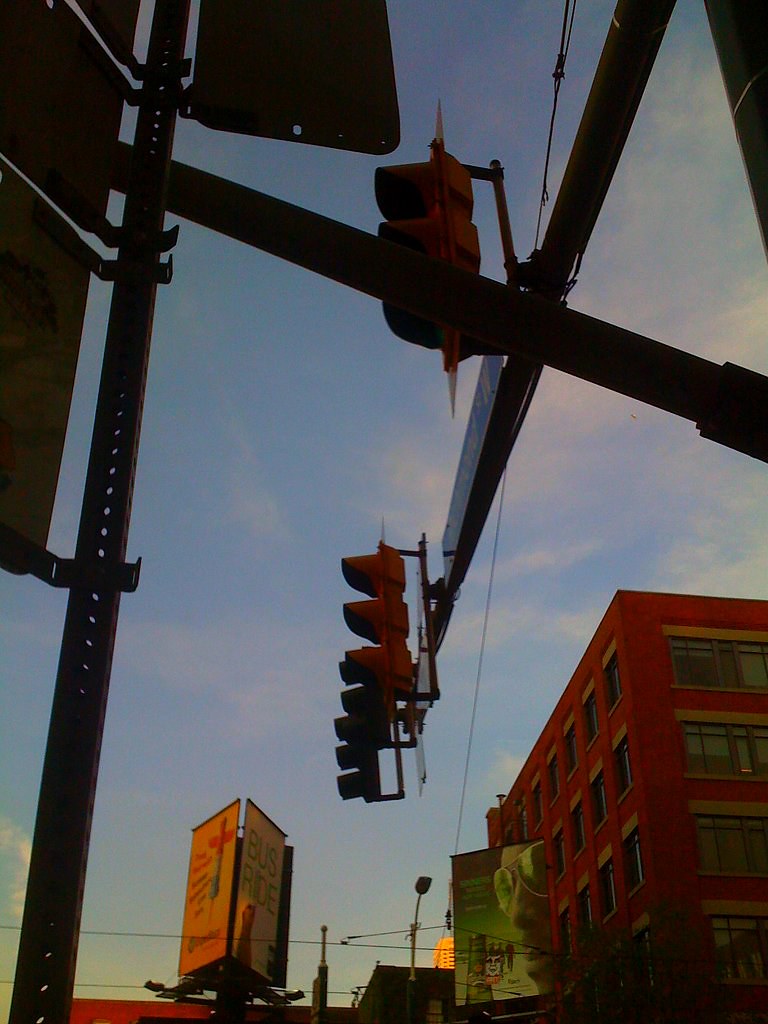This is a real-life photograph of an urban street scene captured from a low angle, looking up at traffic lights. The image has a silhouette effect as it was taken around sunset, creating a dramatic contrast between the darkening street elements and the still-visible blue sky with scattered white clouds. Central to the image are three yellow traffic lights positioned at an intersecting pole, silhouetted against the fading light and giving the scene a striking outline. 

To the left of the frame, a metal pole supports various street signs, which are indistinguishable due to the silhouetted lighting. These elements frame the foreground of the photograph. In the background, a prominent four to five-story brick building stands tall, its reddish hue partially visible. The building features four rows of windows, each with approximately six windows per row.

Adding more character to the image are two signs on the building. One sign prominently displays a man wearing sunglasses and holding a bottle, although the text is too small to read. Another smaller sign to the left reads "Bus Ride," while a third sign is present but illegible. The composition effectively captures the essence of an evening in the city, blending architectural details with urban signage under the diminishing light.